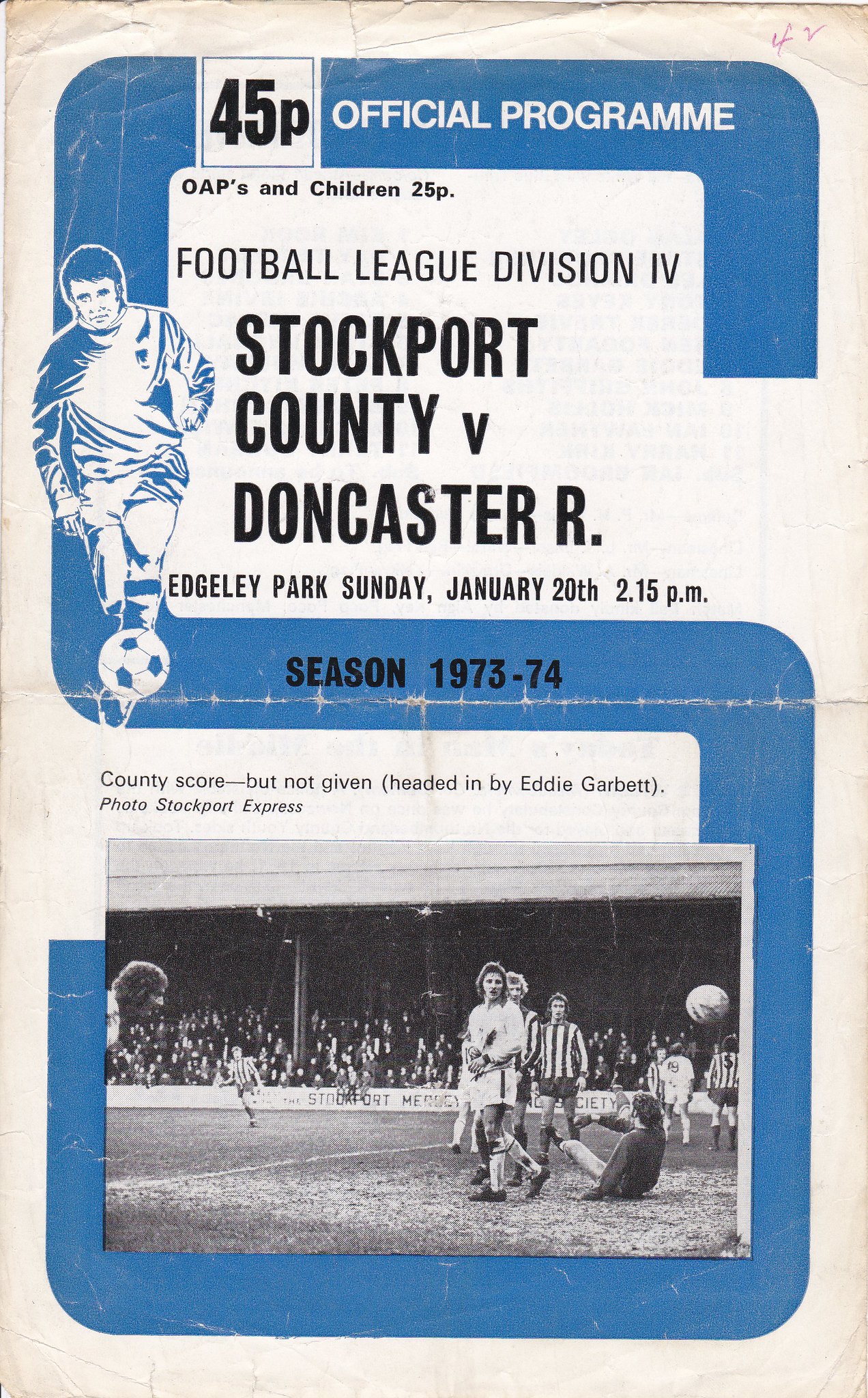The cover of this rugged gameday program, set against a white background, prominently features a large blue "S" that stretches diagonally across the top. In the upper left corner, within a small box, it reads "45P" with "Official Program" written just below. Another piece of text inside the first loop of the "S" indicates, "OAPs and Children 25P." Centered on the cover, bold black text announces, "Football League Division IV, Stockport County vs. Doncaster R, Edgeley Park, Sunday, January 20th, 2.15 p.m., Season 1973-74." The illustration of a soccer player kicking a ball decorates the top left of the cover. Across the middle, it states, "Season 1973-74." Dominating the bottom section is a black and white photograph capturing a dynamic soccer match in progress, with players, referees in black and white striped shirts, and a crowd-filled seating area. Just above this photo, a caption reads, "County score but not given. Headed in by Eddie Garbutt. Photo Stockport Express."